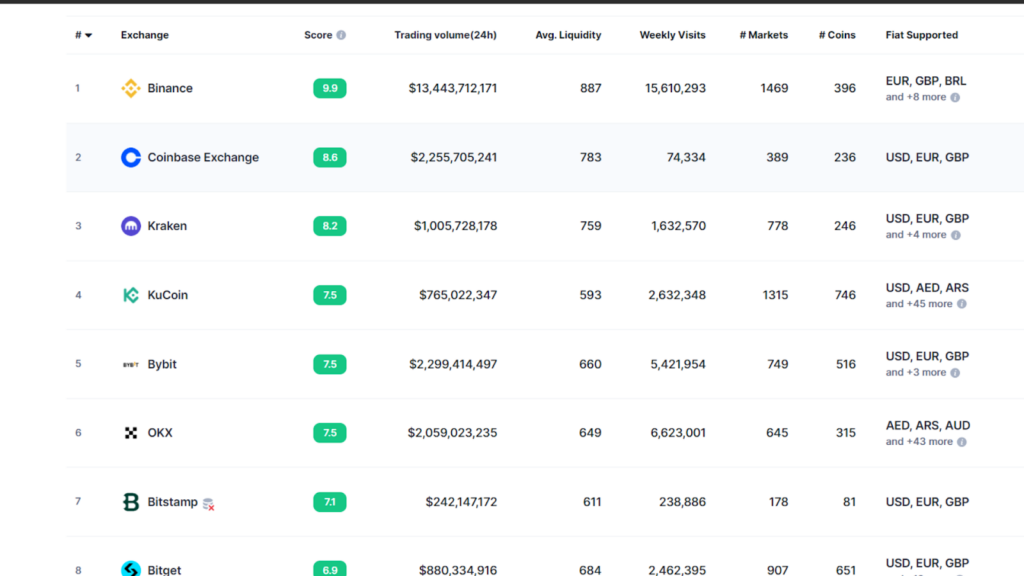A detailed summary of a chart depicting comparative statistics for various cryptocurrency exchanges, indicating their rankings, scores, and other performance metrics such as trading volume, average liquidity, weekly visits, number of markets, and supported fiat currencies. 

At the top of the chart, various criteria are listed, including "Exchange Score," "Trading Volume (24h)," "Average Liquidity," "Weekly Visits," "Number of Markets," and "Number of Coins/FIAT Supported."

1. **Binance** holds the first position with an impressive exchange score of 9.9.
2. **Coinbase Exchange** comes in second with a score of 8.6.
3. **Kraken** ranks third, boasting a score of 8.2.
4. **KuCoin** secures the fourth position with a score of 7.5.
5. **Bybit** also achieves a score of 7.5, tying with KuCoin for the fourth position.
6. **OKX** ranks similarly with a score of 7.5.
7. **Bitstamp** follows with a score of 7.1.
8. **Bitget** rounds out the list with a score of 6.9.

In addition to these scores, each exchange lists metrics like their 24-hour trading volume, average liquidity, weekly visits, number of markets available, and the count of supported cryptocurrencies and fiat currencies. This comprehensive chart offers a detailed comparison for potential users to evaluate the performance and offerings of prominent cryptocurrency exchanges.